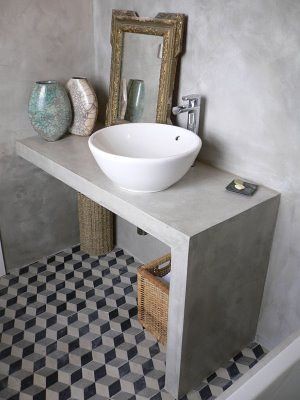A beautifully composed photograph captures a charming rustic bathroom setup. At the forefront, a pristine white ceramic basin with a sleek silver faucet elegantly sits atop a gray, angled wooden stand. Above the basin, a small mirror with an old, rustic brown frame adds a touch of vintage charm to the scene. Flanking the basin are two pottery pieces resembling vases, although both stand empty.

Beneath the angled wooden stand, two distinct baskets rest on the patterned floor; one tall and cylindrical, no more than a foot in diameter, and the other a square wicker basket containing some visible linen, likely towels. The floor itself boasts a captivating pattern of diamond-shaped tiles, creating a 3D optical illusion that enhances the overall aesthetic of this quaint and cozy space.